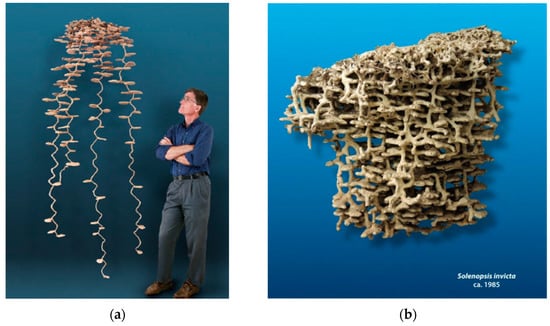The images showcase two side-by-side photographs labeled A and B, set against a blue background. Both images depict intricate structures, most likely anthill castings, revealing the subterranean chambers formed by ants. Image A, on the left, shows a man standing beside a sprawling, tree-like metal sculpture with extended, stringy tendrils that evoke an underwater scene of waving kelp or coral. This sculpture likely results from pouring molten metal into an anthill, illuminating the extensive network of tunnels and chambers beneath the ground. Image B, on the right, presents a more compact version of the casting, labeled with the scientific name "Solenopsis Invicta circa 1985" in white text on the lower right side. This casting is denser and less sprawling than the one in Image A, providing a stark comparison of how different ant species, or environmental conditions, affect the structure of their underground homes. The detailed representations capture the complexity of ant architecture and highlight the diversity in their subterranean engineering.